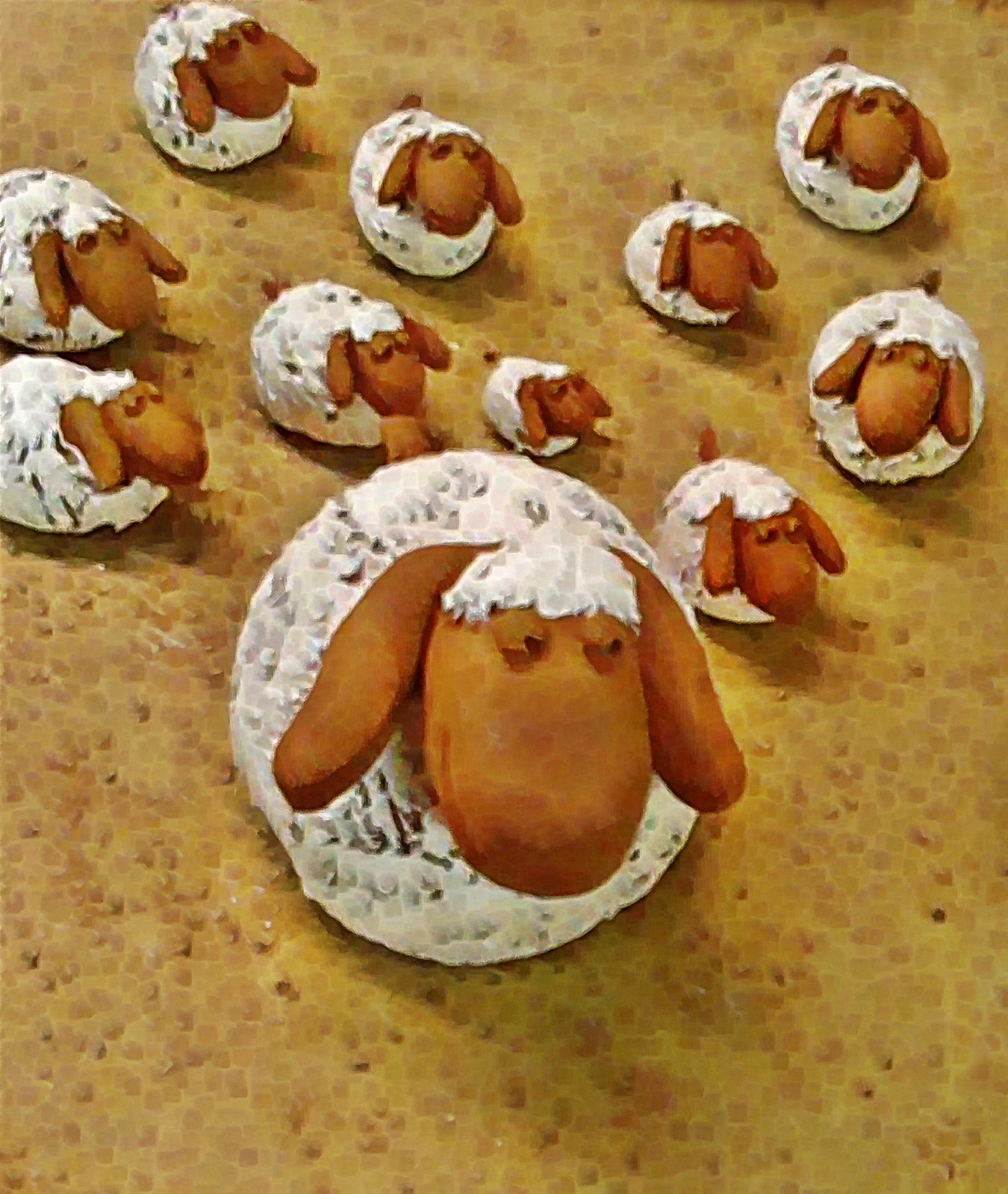This image features a collection of handcrafted clay sheep, reminiscent of characters from a claymation show. The sheep are arranged on a surface that resembles pebbled, orange-brown material with small dots, akin to skin with pores or a textured cobblestone.

At the forefront stands the largest sheep, composed of a big, round white play-doh body. Attached to the body is a brown clay head with two long brown ears, adorned with a tuft of curly white play-doh on top. The face is characterized by two small eyes and a wide, endearing smile.

Scattered behind the main sheep are nine additional sheep of varying sizes—from adult-sized to small "baby" sheep. These smaller sheep maintain the same design, featuring white clay bodies with brown heads and ears, all sporting the iconic white puff on top.

The arrangement of the sheep is as follows: two to the left and two to the right behind the largest sheep, with another one located in the upper left-hand corner. There are five more sheep interspersed among these, creating a delightful scene of diverse, whimsical characters.